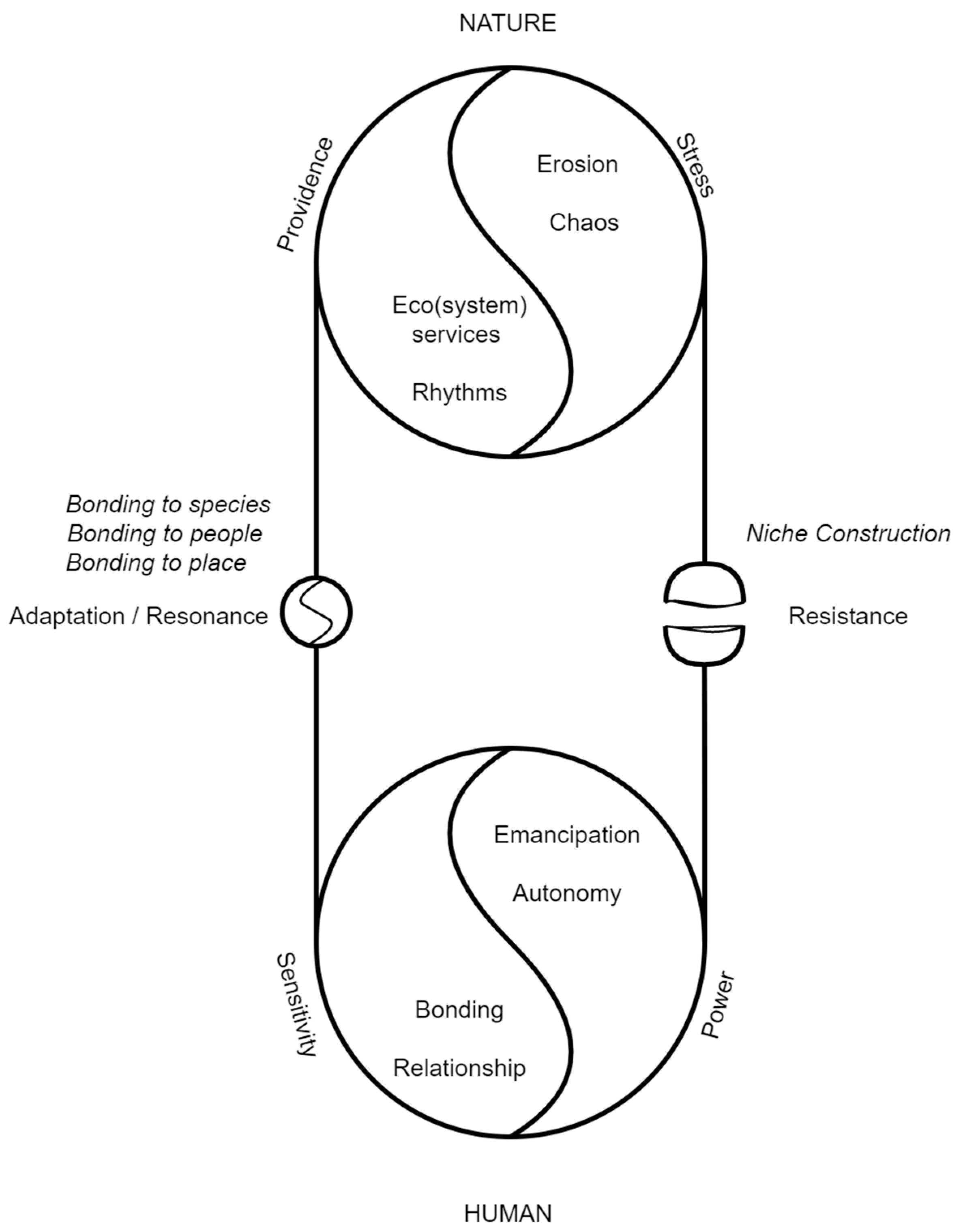The image is a detailed black-and-white diagram with two large yin-yang-like circles connected by lines, set against a solid white background. The top circle is labeled "Nature," and the bottom one is labeled "Human." Each circle is divided into two halves and features distinct keywords. In the Nature circle, "providence" and "stress" flank the surface, with "erosion" and "chaos" on the right interior, and "ecosystem services" and "rhythms" on the left. The Human circle has "sensitivity" on the left and "power" on the right, with "emancipation" and "anatomy" inside, and "bonding" and "relationship" on the left. Additional text surrounds and connects the circles, including terms like "adaptation," "resilience," "niche construction," "resistance," "reunification," "economy," "connectivity," and "scalability." This complex visualization appears to examine the interrelation and comparison between natural and human elements, possibly intended for educational purposes.